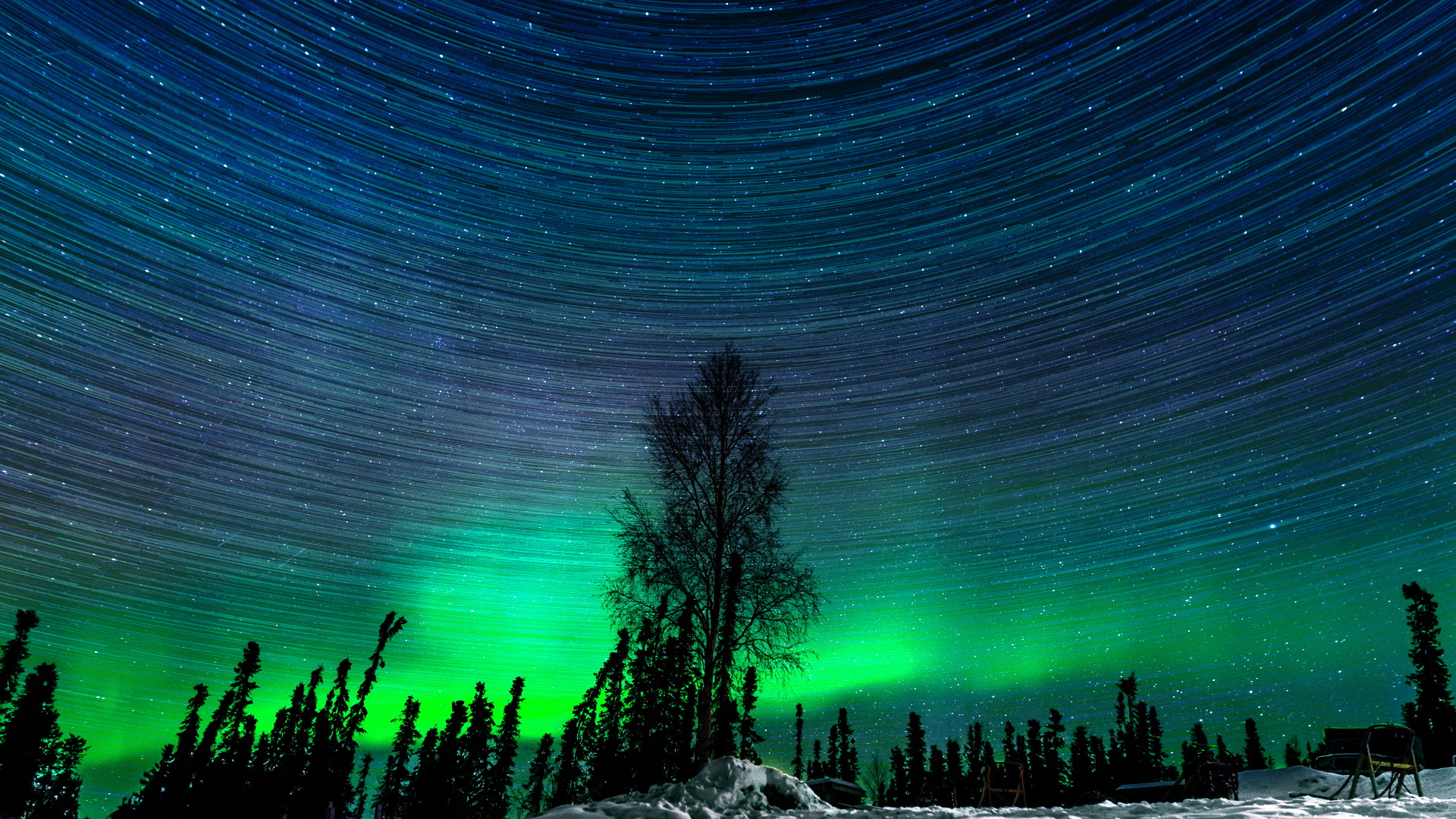This image is a mesmerizing long-exposure night scene, capturing a stunning view of the northern Arctic landscape. The sky, the focal point of the composition, is filled with circular streaks of stars, creating a surreal, almost capsule-like effect. These trailing lines blend beautifully with the vibrant hues of blue and green, similar to the aurora borealis, which glow intensely, especially at the horizon's center. Thin, small pine trees populate the foreground, standing over patches of snow and rocks, adding to the scene's pristine and chilly atmosphere. The sky boasts an array of stars and occasional clouds, hinting at the depths of the Milky Way. The combination of these elements creates a breathtaking, dreamlike depiction of a night in the Arctic wilderness.